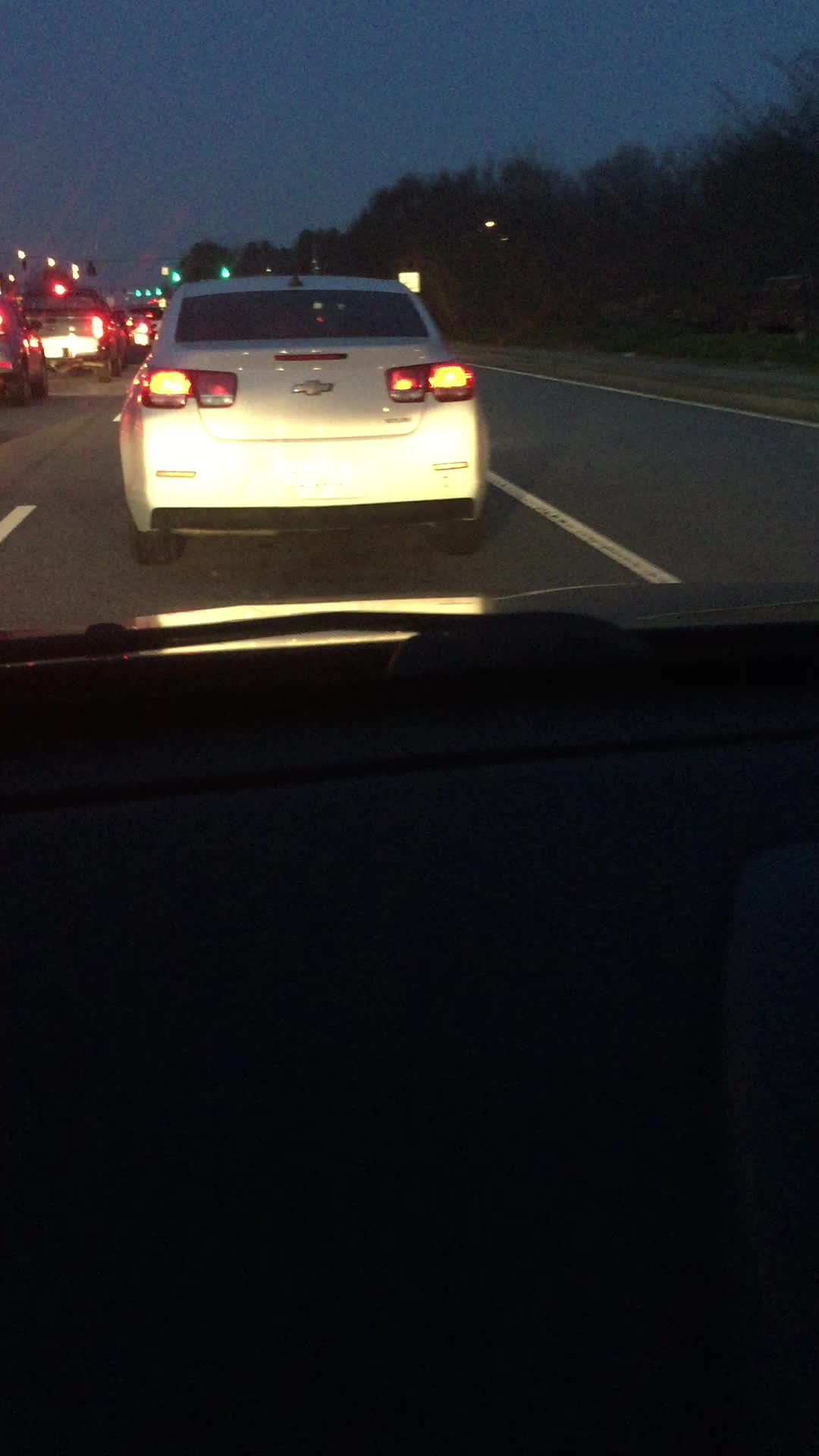A vertical rectangular nighttime image captures the view from inside a car on a multi-lane highway. Through the windshield, a cream-colored Chevrolet with illuminated taillights is prominently visible. The Chevrolet's symbol glows faintly, reflecting the headlights. Traffic appears at a standstill, as all vehicles have their brake lights lit, indicative of slow-moving congestion possibly due to a far-off intersection or traffic backup. In the upper left corner, a traffic light subtly hints at stop-and-go conditions. To the right, there is a line of trees and an additional, seemingly open lane. A road sign is visible beside the Chevrolet. The sky is a dark gray, softly illuminated by the ambient city lights, encapsulating the scene of sitting in traffic at night, waiting to progress forward.